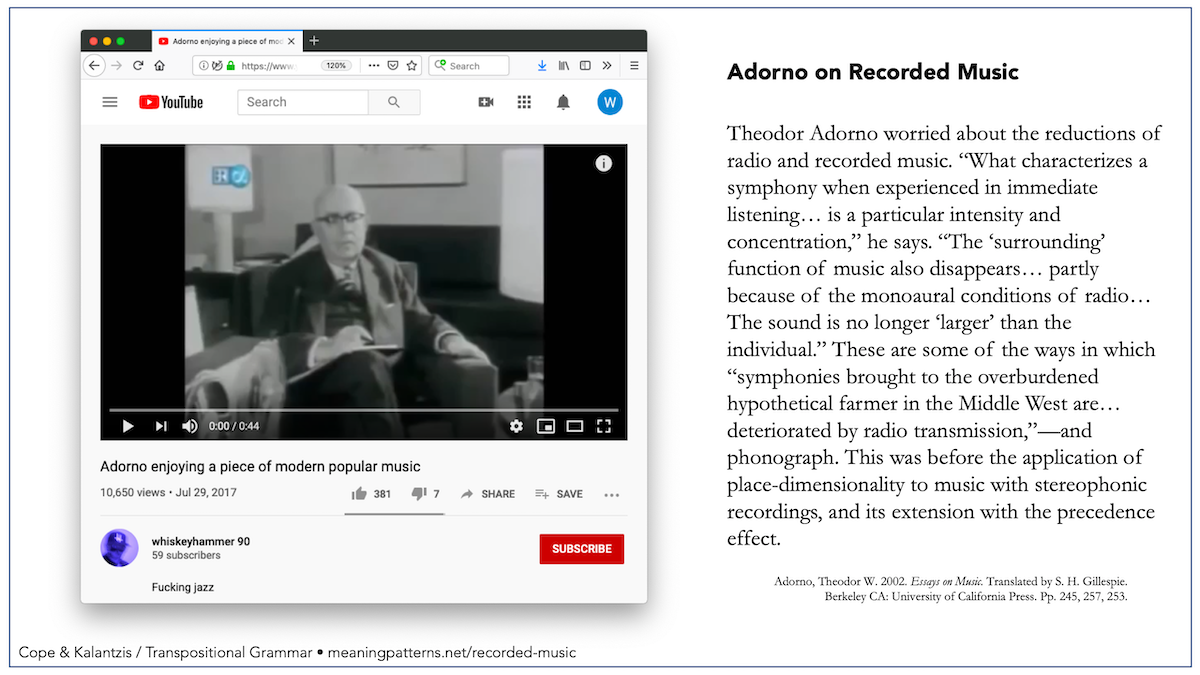This image features a bordered frame. Within this frame, on the left side, there is a screenshot of a YouTube video titled "ADORNO." The video discusses the drawing of modern popular music by Adorno. The visuals in the clip are in black and white, depicting a bald man seated on a chair, with a notebook resting on his knee. He is gazing forward and wears black-framed glasses. The video has accumulated 10,650 views and was posted on July 29, 2017. It has received 381 likes and 7 dislikes. On the right side of the image, there is text that reads "ADORNO on recorded music." Below this heading, there is a paragraph of text followed by smaller writing.